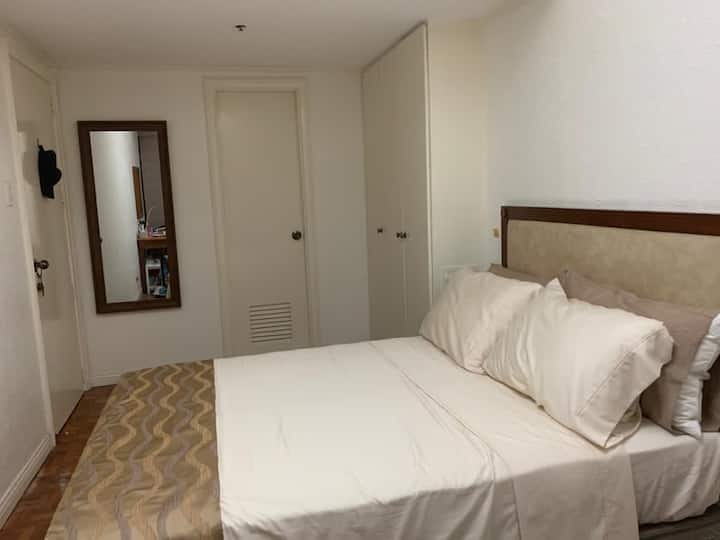This photograph depicts a spacious hotel room featuring predominantly white walls and a tan baseboard with a brown rim. Central to the image is a large bed, oriented horizontally within the frame and occupying most of the room. The bed is adorned with a mix of white and brown pillows—the white pillows stacked against the headboard and the brown pillows positioned in front of them. The bedding consists of crisp white sheets with a detailed brown and tan patterned bedspread at the foot of the bed. 

The bed’s headboard is a padded wooden frame upholstered in a light tan fabric. Directly in front of the bed is a white door, presumably leading to the bathroom. To the right of this door is a cabinet, and on the left is a full-length mirror bordered with brown wood. Adjacent to the mirror, towards the left side of the room, is another door with a piece of cloth hanging from it, likely leading to a closet or the room's exit. The room's plain yet elegant decor is accentuated by the clean lines and minimalistic design elements that contribute to its serene ambiance.